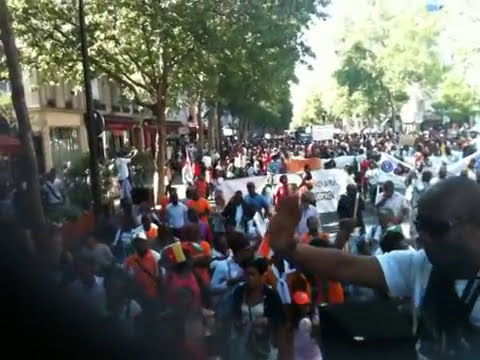This photograph captures a vibrant rally or demonstration on a road, completely filled with people. The diverse crowd, primarily black-skinned individuals, are holding various signs and banners, many of which are bright orange and white. Near the forefront of the image, a bald man in sunglasses and a white shirt, possibly carrying a black backpack, directs his attention to the left. The scene is bordered by trees with green leaves and brown trunks, creating a natural frame for the event. Beyond the trees, in both the top left and top right corners, there's a row of red, tan, and green buildings that line the street, providing an urban backdrop to the bustling activity below. The image is colorful with people in different attire, highlighting the collective energy of the gathering.